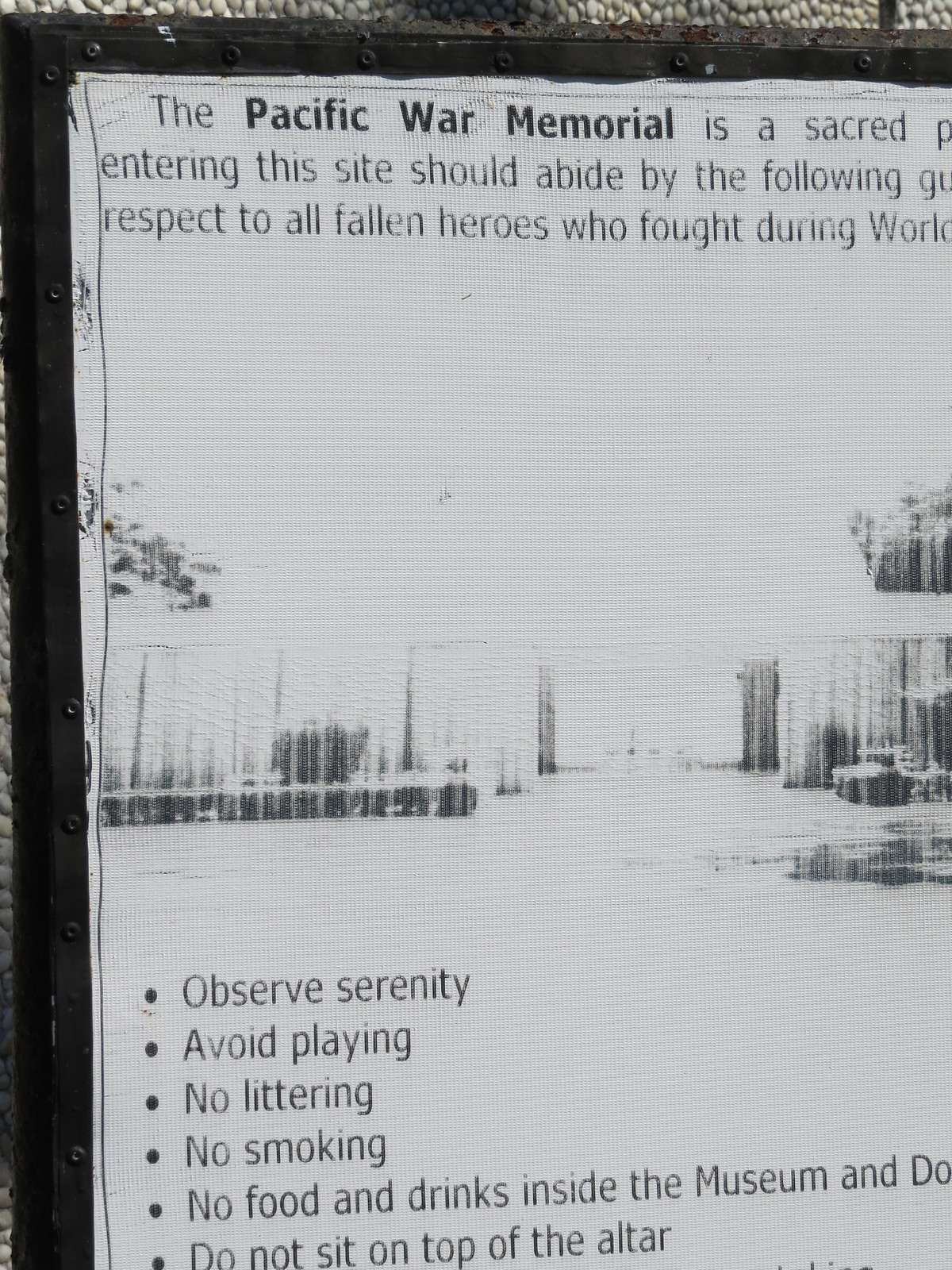The black and white image depicts an outdoor scene focused on an old, weathered sign against a stone wall at the Pacific War Memorial. The sign's text, slightly cut off at the edges, communicates a reverent message: "The Pacific War Memorial is a sacred site. Entering this site should abide by the following guidelines: Respect to all fallen heroes who fought during World War II. Observe serenity. Avoid playing. No littering, no smoking, no food and drinks inside the museum. Do not sit on top of the altar." The photograph, of low quality, makes it difficult to distinguish details clearly, but the image appears to be taken during the day and shows hints of surrounding trees or foliage. The colors are limited to shades of white, black, and gray, and the sign dominates the composition, filling almost the entire frame while appearing slightly cut off at the edges.